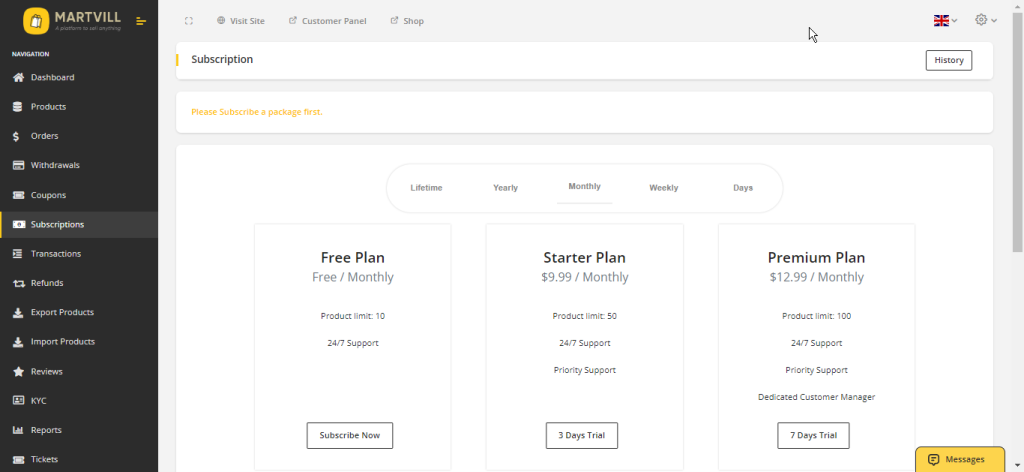This is a landscape-oriented screenshot from a PC, featuring a partial capture of a software named "Martville." On the left side, there is a vertical menu section with a dark grey, almost black background and white text. The menu lists various options: "Dashboard," "Products," "Orders," "Withdrawals," "Coupons," "Subscriptions," "Transactions," "Refunds," "Export Products," "Import Products," "Reviews," "KYC," "Reports," and "Tickets," each accompanied by an appropriate icon to their left. The "Subscriptions" option is highlighted. At the very top of this menu is the word "Martville" in white text, next to a small, yellow, rounded square containing a white shopping basket icon.

The main body of the page has an off-white, greyish background with white content boxes. The top border features navigation options: "Visit Site," "Customer Panel," and "Shop," each with corresponding symbols. The top right corner displays a British flag and a settings cogwheel. Below this is a long, rectangular section with black text, labeled "Subscription" on the far left and "History" on the far right. Underneath, a slightly smaller rectangle with dark yellow text states, "Please Subscribe and Package First," separated by a small divider.

The rest of the page is dedicated to showcasing different subscription plans, divided into three columns labeled "Free Plan," "Starter Plan," and "Premium Plan." 

- The "Free Plan" column includes the text "Free / Monthly," with additional details in smaller text: "Product Limit 10," and "24x7 Support." A small box below it reads "Subscribe Now" with a black text on a white background.
- The "Starter Plan" column is priced at "$9.99 Monthly," followed by details: "Product Limit 50," "24x7 Support," and "Priority Support." An adjacent box offers a "Three Days Trial" in black text within a white box with a black border.
- The "Premium Plan" is priced at "$12.99 Monthly," with smaller text specifying: "Product Limit 100," "24x7 Support," "Priority Support," and "Dedicated Customer Manager," each on separate lines. It also features a "Seven Days Trial" box with a black border.

In the bottom right corner of the image, there is a small yellow box with the word "Messages" in black text, alongside a message icon.